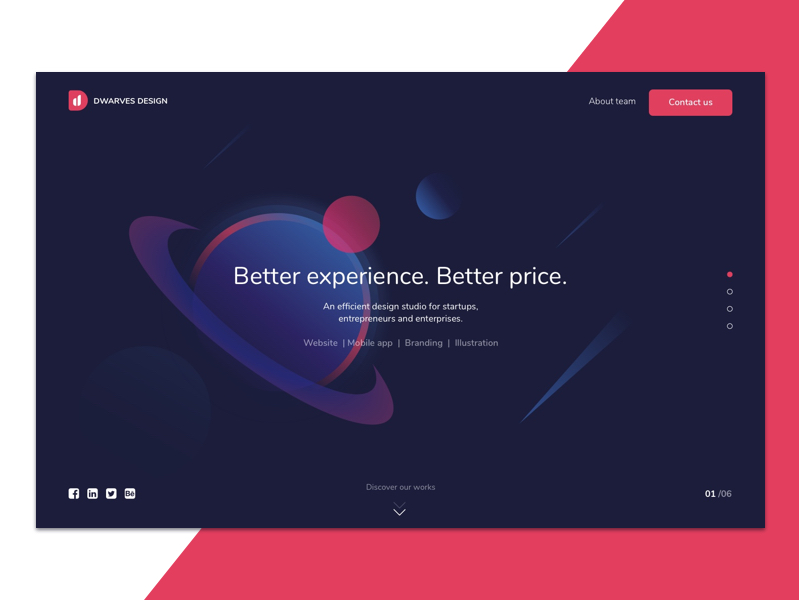This intricate design is crafted by Dwarbus Design, whose logo features a distinctive pink 'D' with two vertical lines intersecting it. The layout is quite sophisticated. Envision a solid navy blue box set against a partially pink background that extends for about two inches and is diagonally cut, allowing only this segment to appear behind the navy box.

Within the navy box, the focus is on their "About Team" section. Adjacent to this, set within the pink portion, is the "Contact Us" section. Additionally, there is a depiction of Saturn, complete with its rings, surrounded by smaller planetary objects.

The text reads, "Better experience, better price. An efficient design studio for start-ups, entrepreneurs, and enterprises," emphasizing their core services which include website design, mobile app development, branding, and illustration.

Accenting the composition are a couple of light blue swishes. Towards the end of this page, it is noted as the first of six, featuring an invitation to "Discover our works" along with a downward arrow, guiding the viewer to explore further.